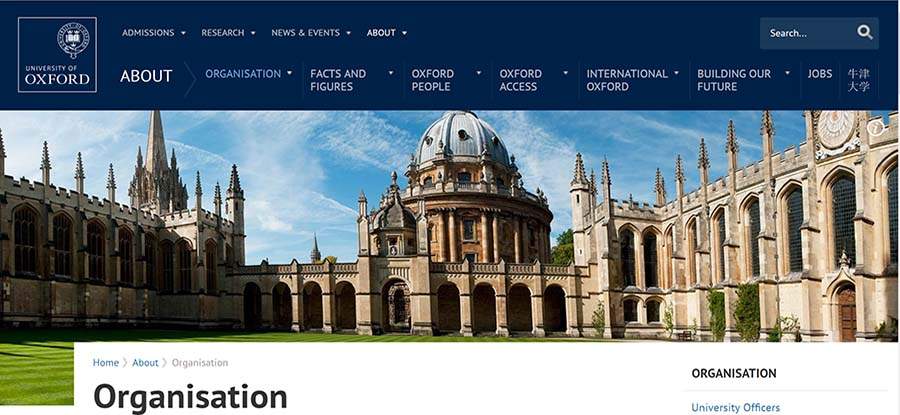The image depicts the homepage of the University of Oxford's website. In the top left corner, within a white box, the name "University of Oxford" is displayed in white text. Positioned above this, slightly to the right, is a small logo consisting of a circle with a bird at the bottom. Adjacent to the logo and a bit higher up, four primary navigation categories are listed: "Admissions," "Research," "News and Events," and "About."

Beneath this navigation bar, there are additional categories presented in a larger font: "About," "Organization," "Facts and Figures," "Oxford People," "Oxford Access," "International Oxford," "Building Our Future," and "Jobs." At the very top right of the image, a small boxed area contains the word "Search" in white text followed by an ellipsis, with a magnifying glass icon located to the far right within the same boxed area.

The central portion of the image features a photograph of the university, showcasing a large building centrally located and extending sideways, bordered by an expansive grass field below it. To the bottom left of the image, the word "Organization" is prominently displayed in large black text, while the bottom right features the phrase "University Officers."